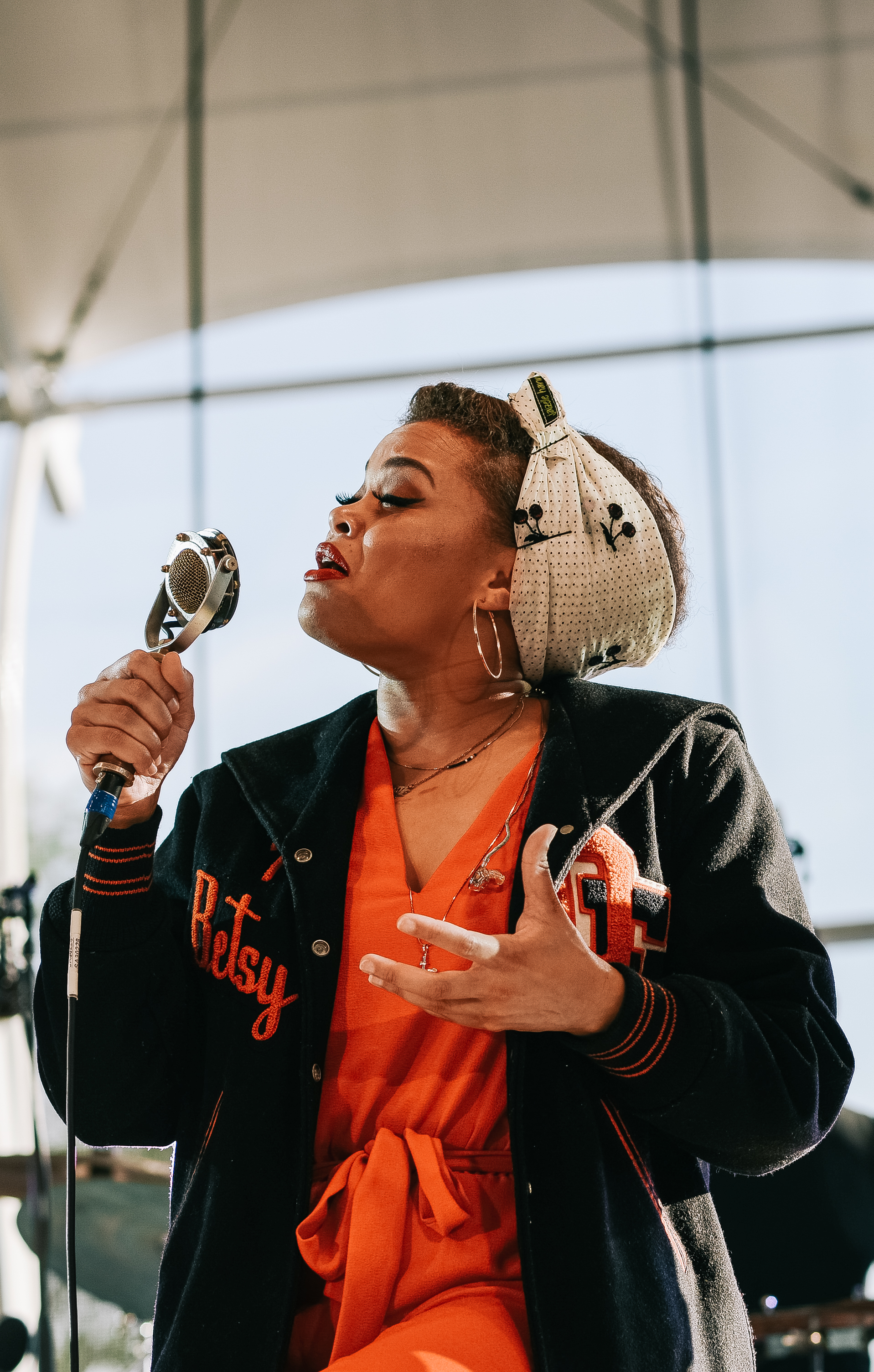The photograph captures an elegant moment of a black woman singing into a retro-style, metallic silver microphone, facing slightly to the left. Radiating energy, she is dressed in a stylish black wool sports jacket with the name "Betsy" prominently embroidered in orange cursive on the left side, and likely more letters on the right side that are not visible. The ensemble is complemented by an orange v-neck shirt tied at the front and matching orange pants. Her accessories include large silver hoop earrings and a neatly tied black and white polka-dotted headscarf securing her curly hair. The woman is identified as possibly being Jill Scott, characterized by her radiant red lipstick and expressive singing stance, with her left leg slightly lifted and her left hand open. The background reveals she is performing at an outdoor venue with an open sky tinted light blue, marked by scaffolding and structures holding up a tall ceiling, suggesting a daytime event. Some musical instruments can be spotted on the ground floor behind her, reinforcing the scene’s dynamic atmosphere.